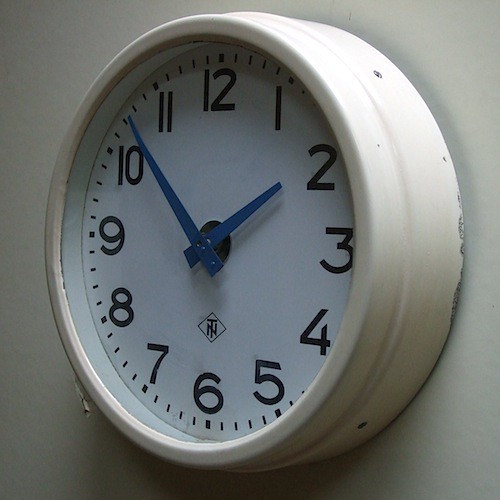The image displays a wall clock with a metal exterior, featuring a rounded and somewhat thick design. The clock is mounted on a smooth, white-painted drywall surface. Its face is white, adorned with black numerals from 1 to 12, with the number 12 positioned at the top. Both the hour and minute hands are strikingly blue, adding a touch of color to the monochromatic scheme. There is also a distinctive logo on the clock, resembling a diamond shape with the letters "N" and "T" intersecting within it, though the specific brand remains unidentified. The clock's face also includes thick dashes marking each hour and smaller dashes in between for minute intervals, adding to its detailed and functional design.